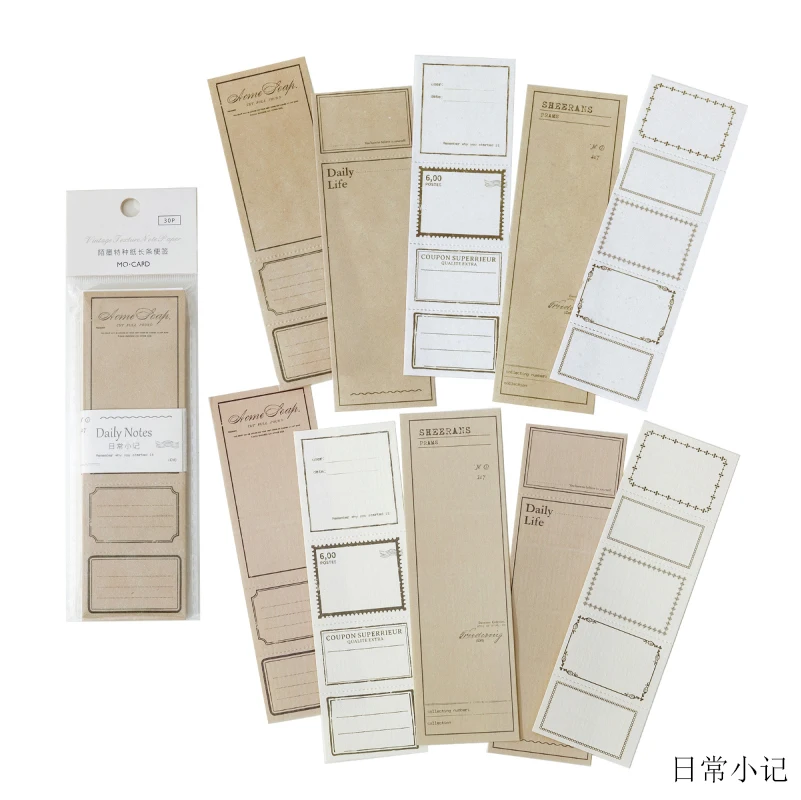The photograph showcases a collection of Asian stationery products, predominantly featuring a neutral color palette of whites, golds, and natural paper browns against a stark white background. Centered prominently is a pack containing 30 pieces, including various stickers and post-it note-style papers, indicative of their utility for letter writing, note-taking, or journaling. Adjacent to the pack, there are several long, rectangular gift tags exhibited both individually and within branded packaging, hinting at the possibility of them being sold on a specialized website. The consistent use of kanji across the items suggests their origin as either Japanese or Chinese. The packaging displays categories like "daily notes," "coupons," and "beauty," with each piece featuring neat borders and an organized layout of text and designated writing areas.